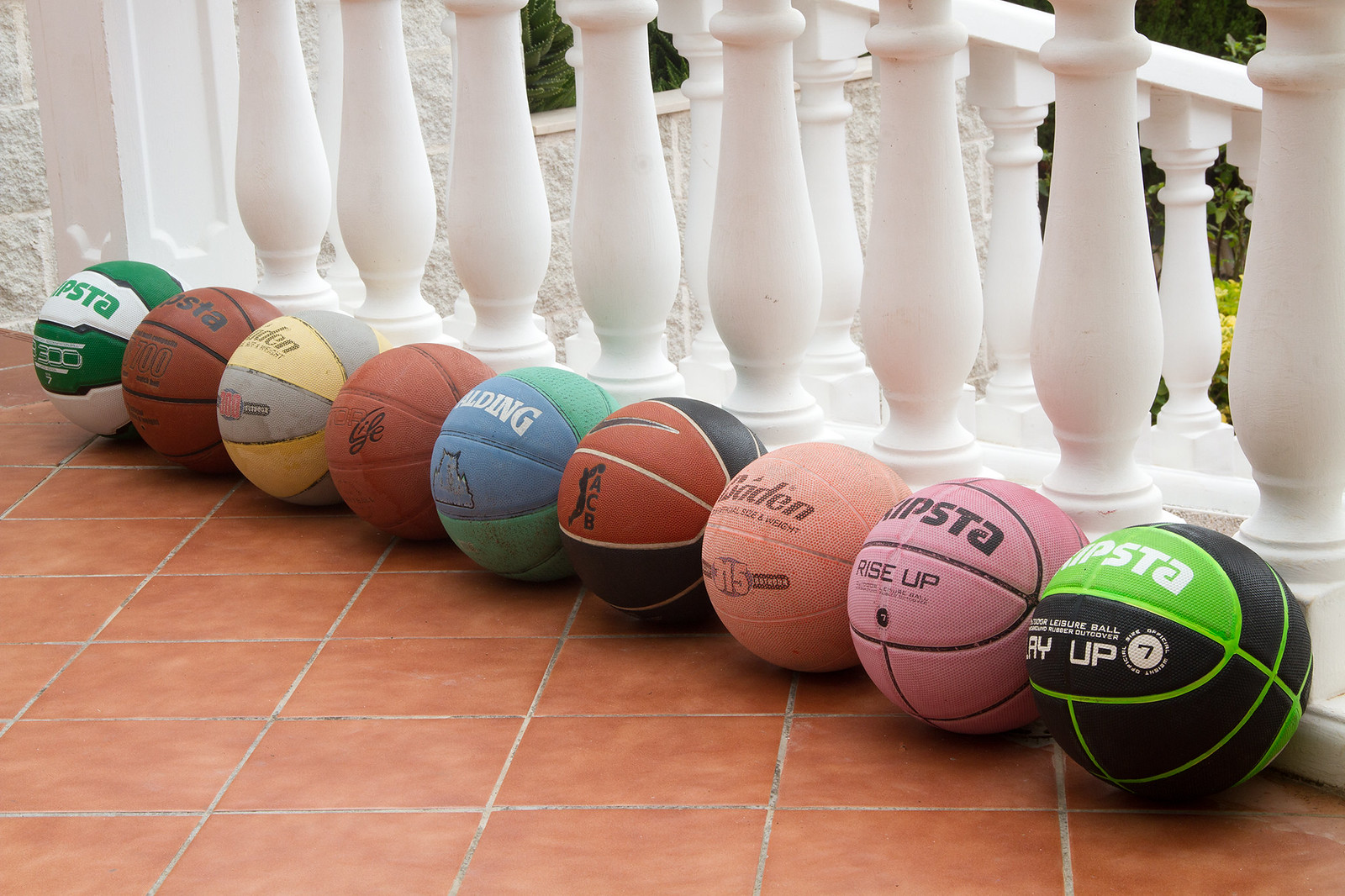This is a detailed color photograph taken outdoors during the daytime. The image captures a neat and artistic scene where nine basketballs are lined up diagonally on a porch made of terracotta-colored square tiles with visible grout lines. The basketballs, all uniform in size but varying in color, are arranged as follows: starting from the left, the first is green and white, followed by a dark orange one, a yellow and gray ball, another dark orange ball, a blue and green ball that appears to have the word "Spalding" on it, then a burnt orange and black ball, a light orange ball, a pink one, and finally, a black and green striped basketball located closest to the viewer with some indistinct lettering. The porch is backed by a sturdy-looking railing made up of large, white pillars, giving the scene a structured and heavy-duty appearance.